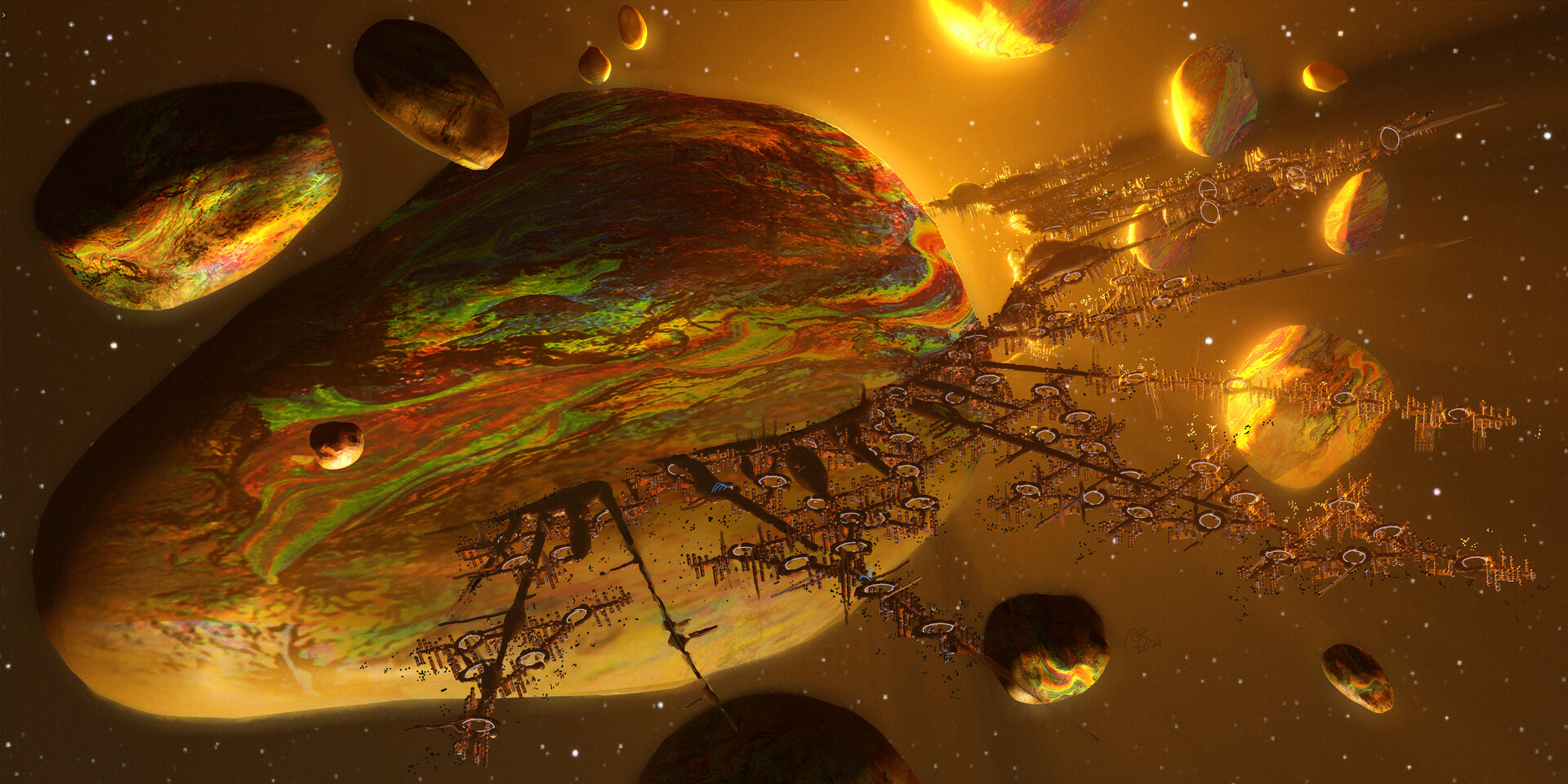This is a highly detailed, computer-generated sci-fi image depicting a celestial scene in space. The primary focus is a gigantic, irregularly shaped asteroid situated in the center, with a unique, multicolored surface pattern reminiscent of the kaleidoscopic effect created when oil mixes with water. This includes swirling hues of green, red, orange, yellow, brown, blue, and black. Surrounding this mammoth asteroid are numerous smaller asteroids, each similarly adorned with vibrant, reflective colors due to the luminous Sun partially obscured by the central mass.

Radiating from the main asteroid are numerous branches or rod-like structures, resembling tree limbs. These branches extend outward and hold small, circular pods with black borders, suggesting a semblance of a space colony or complex antennas. The entire scene features a dark, starry sky with dots of white stars creating a speckled backdrop. The vivid interplay of color and light, along with the intricate structures, lends an otherworldly and cosmic ambiance to the image, making it a striking representation of a space landscape filled with both natural and seemingly artificial elements.